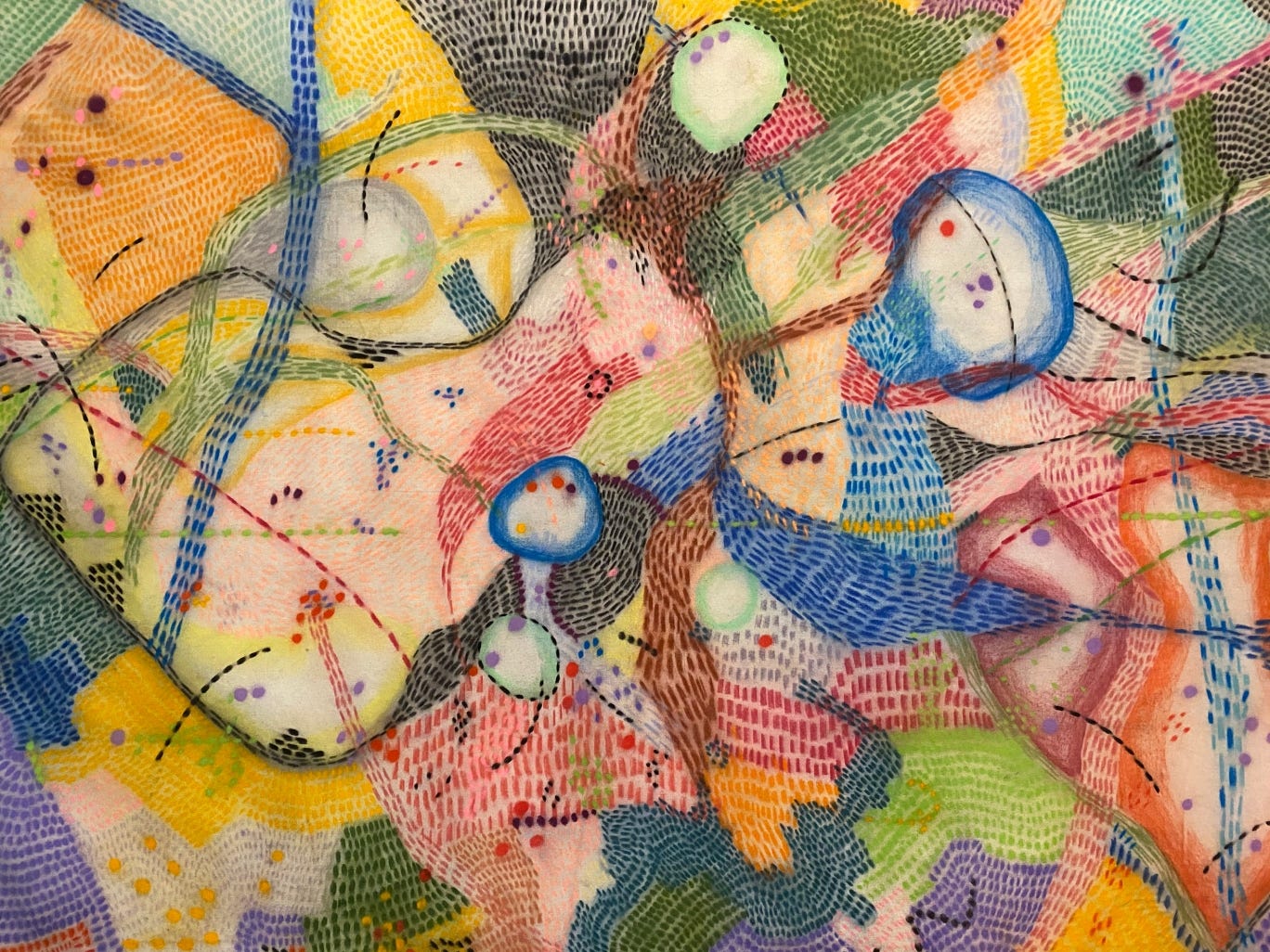The image features abstract art, characterized by an intricate and diverse composition of shapes and colors. It consists of numerous little lines and dots, arranged in groups without repeating patterns, covering the entirety of the piece. The artwork is vibrant and dynamic, incorporating a wide spectrum of colors including black, yellow, blue, light blue, orange, pink, brown, maroon, mauve, lime green, and purple. The shapes within the composition are varied, including round, triangular, and blob-like forms. Some areas are densely colored while others are more sparse. The piece could be interpreted in multiple ways: as a map, a fabric print, or even as stitching. There are elements resembling faces and mushrooms, with polka dots and brick-like patterns interspersed throughout. This complex and undefined arrangement invites the viewer to let their imagination shape their interpretation of the art.